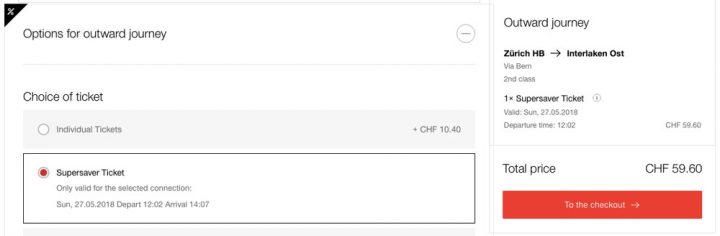**Screenshot Description: Ticket Purchase Screen for Transportation Journey**

The screenshot displays an app or website interface used for purchasing tickets, prominently focused on options for an outward journey. 

**Header Section:**
- At the top, the heading reads "Options for Outward Journey."

**Left Panel:**
- Just below the header, it presents two ticket options:
  - **Individual Ticket**: Priced at CHF 10.40
  - **Super Saver Ticket**: Only valid for the specified connection.
    - Departure: Sunday, May 27, 2018, at 12:02 PM
    - Arrival: 2:07 PM
    - The Super Saver Ticket is selected, as indicated by a red radio button and a black box around it.

**Right Panel:**
- The detailed information specific to the selected Super Saver Ticket is displayed:
  - Departure Location: Zurich HB
  - Destination: Interlaken Ost
  - Route: Via Bern
  - Class: Second Class
  - Ticket Type: One-time Super Saver
  - Date and Time: Consistent with the left panel (Sunday, May 27, 2018, Depart 12:02 PM, Arrival 2:07 PM)
  - Price: CHF 59.60
  - The total price is reiterated to emphasize the cost.

**Bottom Section:**
- At the bottom of the screen, there is a prominent red button labeled "To the Checkout," indicating the next step to finalize the purchase.

This comprehensive setup suggests the user is booking a specific type of discounted transportation ticket from Zurich to Interlaken via Bern.